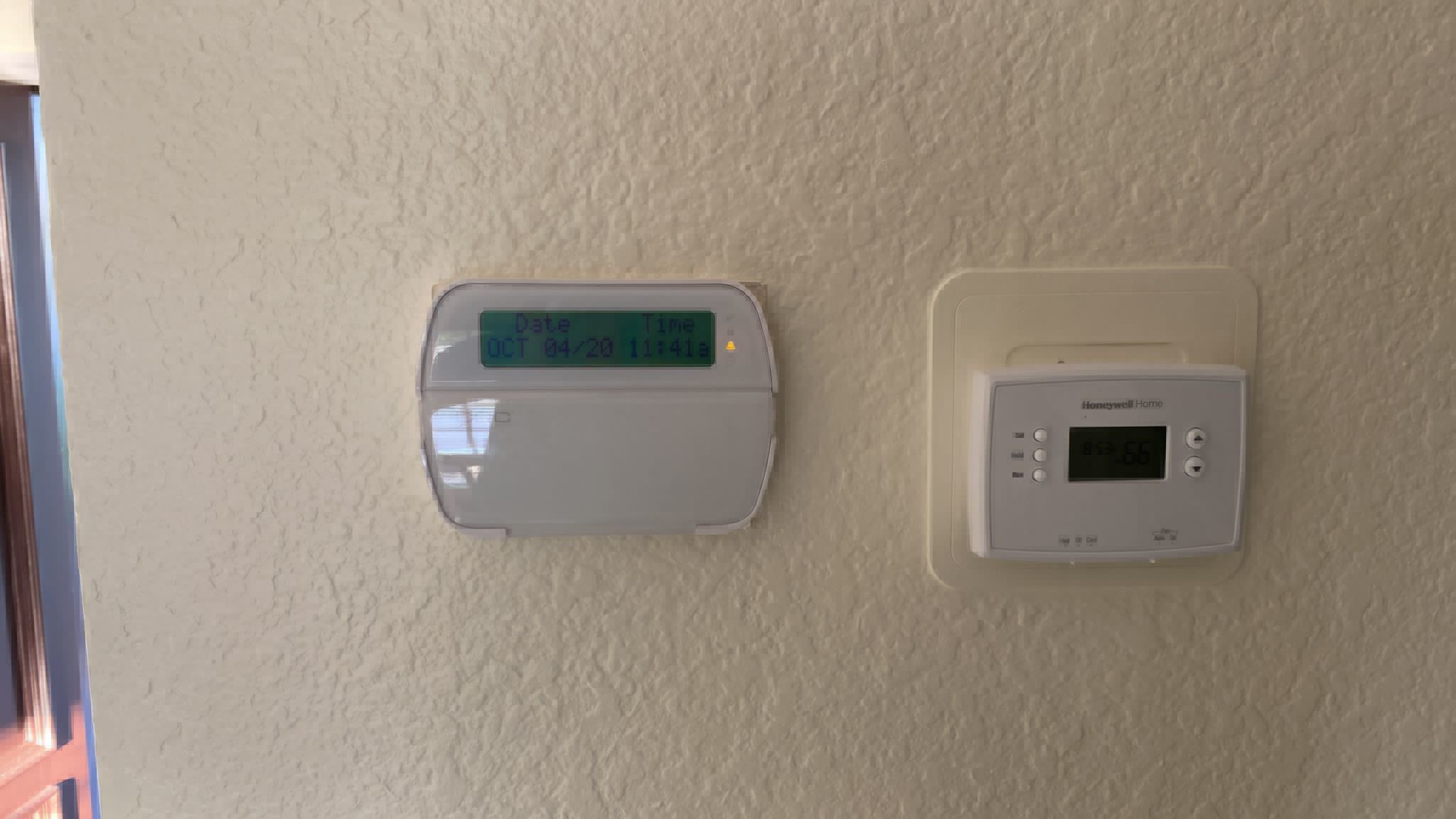This photograph showcases two temperature regulation devices or thermostats mounted on the textured, slightly shiny white wall of a home. Both devices are rectangular, with the one on the left being marginally larger and featuring more curved edges. The screen on the left-hand device displays the date as "October 4th" and the time as "11:41." The right-hand device, which carries the brand name "Honeywell" at its top, appears to be plugged into the wall. This Honeywell thermostat is equipped with three small round buttons on the left and two round buttons on the right, each adorned with black symbols. In the image's left side, the edge of the wall is visible, revealing the corner of another surface. The background of this corner includes a thin, vertically oriented blue object and a horizontally positioned pink object in the lower-left corner.